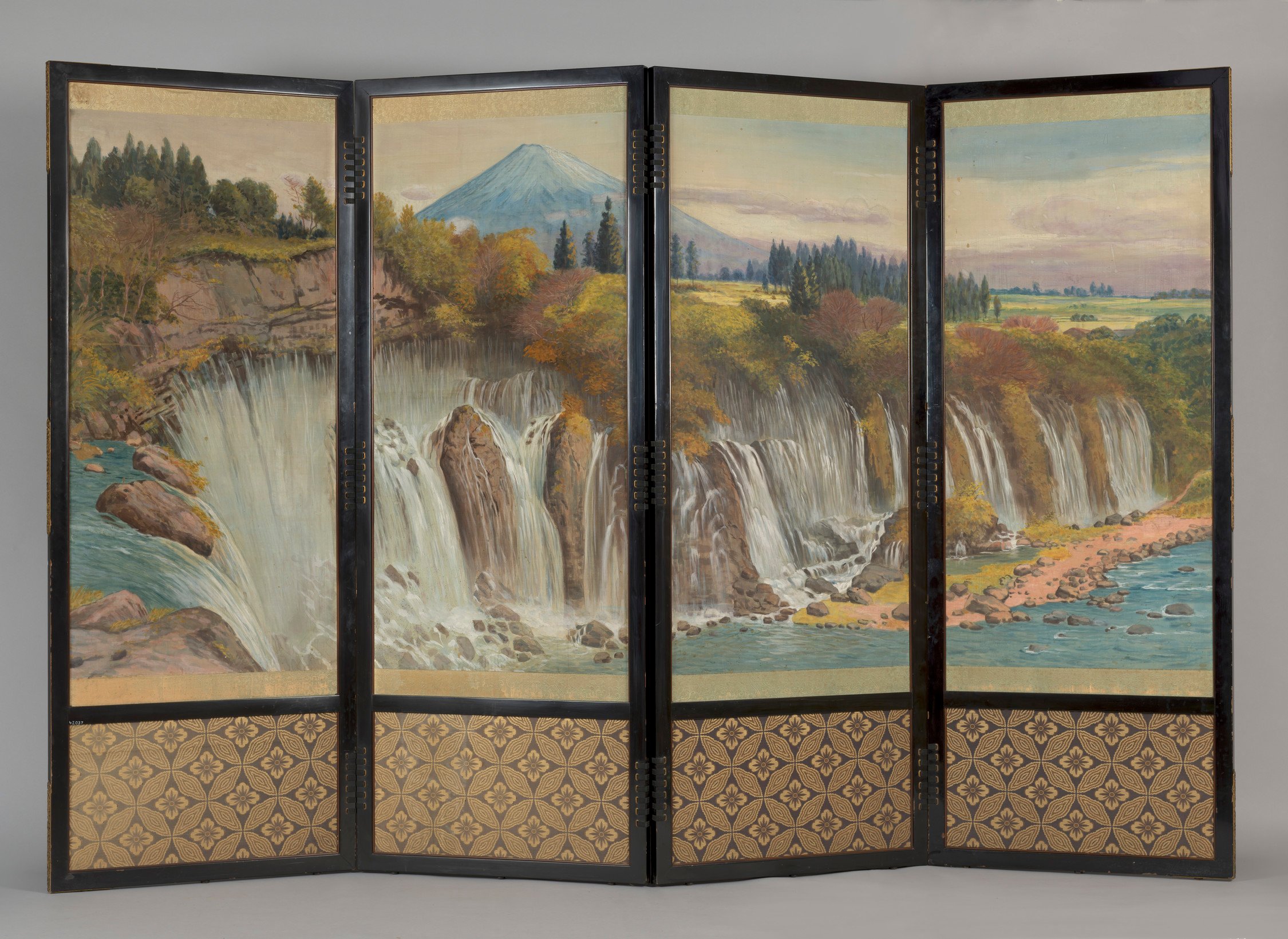This image features an elegant Japanese-style room divider composed of four vertically aligned panels, each connected by black hinges and framed in black wood. The top two-thirds of the panels present a stunning landscape painting depicting a majestic waterfall cascading down a steep cliff with verdant trees and grass adorning its brink. In the far background, the iconic silhouette of Mount Fuji looms, surrounded by sprawling green fields. The bottom third of each panel showcases a brown and tan symmetrical floral design, with darker accents highlighting the flower motifs. The divider stands against a plain cream-white background, further emphasizing its intricate and harmonious artistic composition.